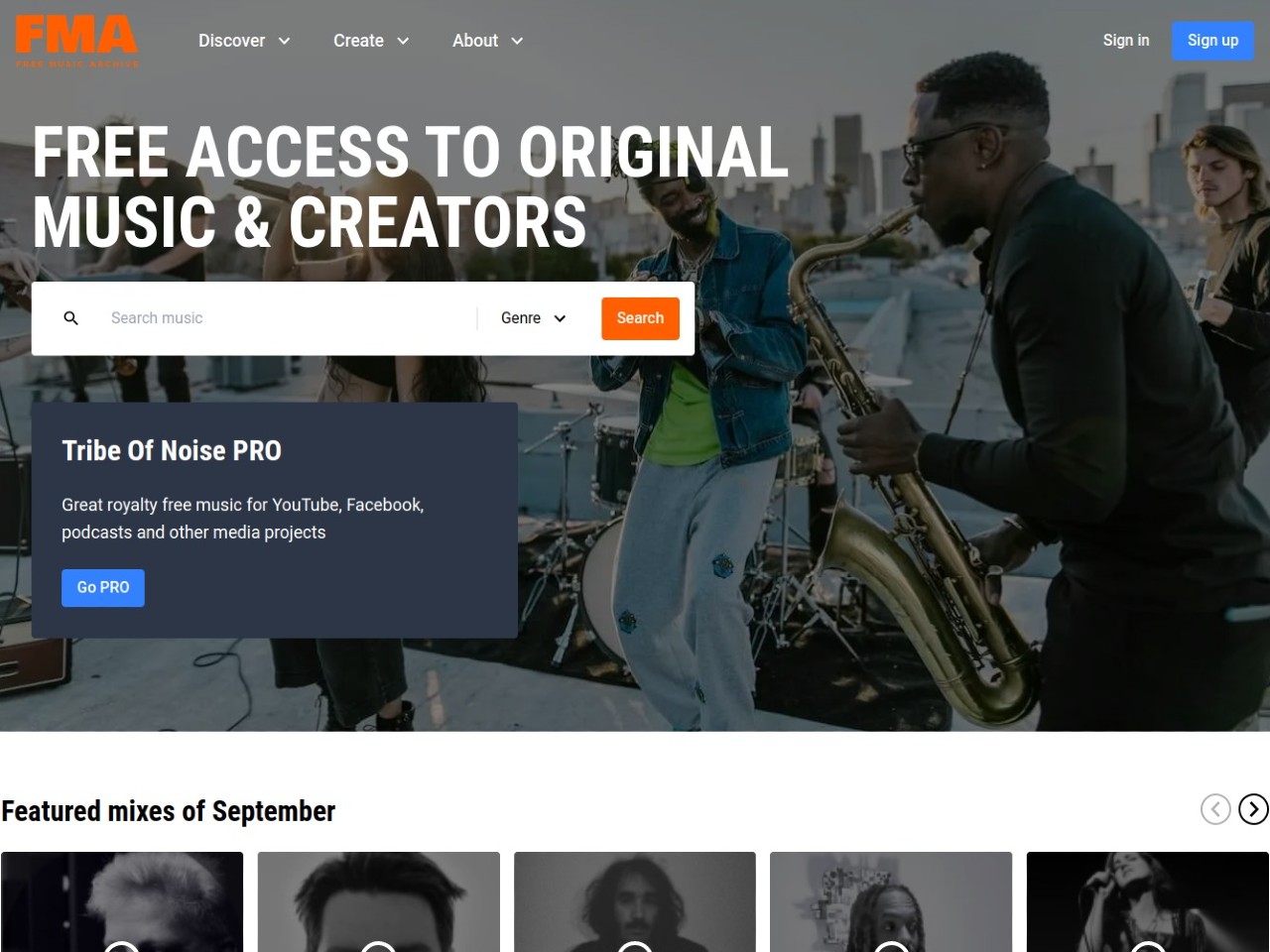The image showcases a webpage layout for FMA (Free Music Archive). At the top left corner, the bold letters "FMA" are prominently displayed. To the right of the FMA logo, there are three navigation tabs labeled "Discover," "Create," and "About," arranged from left to right. In the top right corner of the page, there are two prominent buttons: "Sign In" on the left and "Sign Up" on the right. 

Just below the navigation bar, on the left side, a headline reads "Free Access to Original Music and Creators." Underneath this headline, there is a search bar. Inside the search bar, the placeholder text reads "Search Music." Adjacent to the search bar, there is a "Genre" tab, and next to that, a "Search" button is visible with white text on an orange background.

Further below, there is a section highlighting "Tribe of Noise Pro" with a tagline, "great royalty-free music for YouTube, Facebook, podcasts, and other media projects." Beneath this, a prominent button with white text and a blue background reads "GoPro."

The background of the webpage features an image of people, with a man clearly visible on the right side, playing an instrument. The overall design conveys a user-friendly interface geared towards providing access to free and royalty-free music.